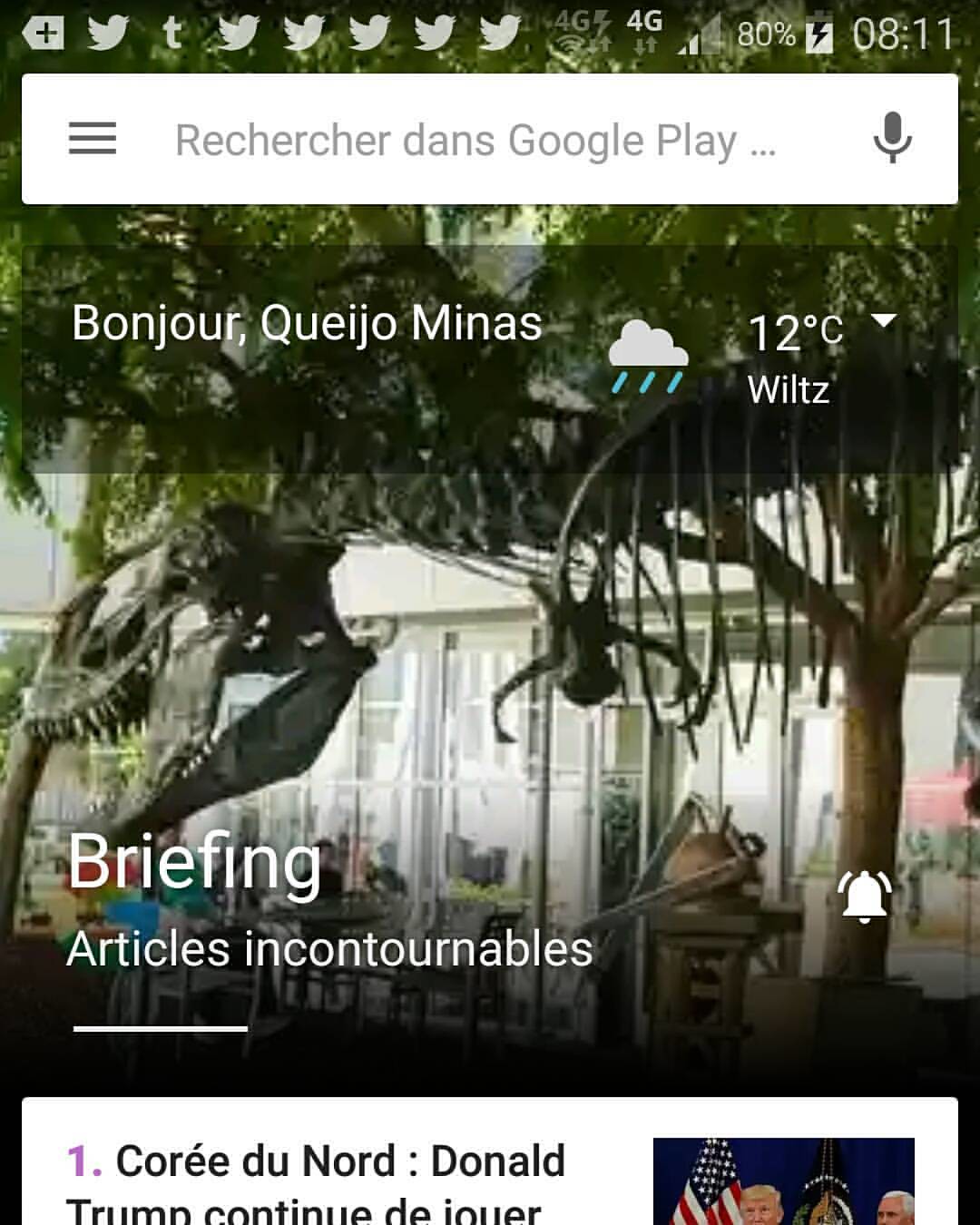The image is a detailed screenshot taken from an Android mobile device, suggesting it might be a cell phone or a tablet. At the top of the screenshot, a series of Twitter notifications are visible alongside a Google search bar. The text appears to be in French, with words indicating weather information, such as "12 degrees Celsius" and potential rain. A timestamp shows 8:11 AM. The background of the screenshot includes images of a downtown area and some skeleton bones, amidst a variety of colors including green, gray, white, black, light blue, dark blue, yellow, red, and purple. The entire image is occupied by this screenshot, emphasizing it was taken from a mobile device. No people are present in the image, but there is a mention of names like Cory, Donald Trump, and juror, likely from a Twitter post or notification within the screenshot.